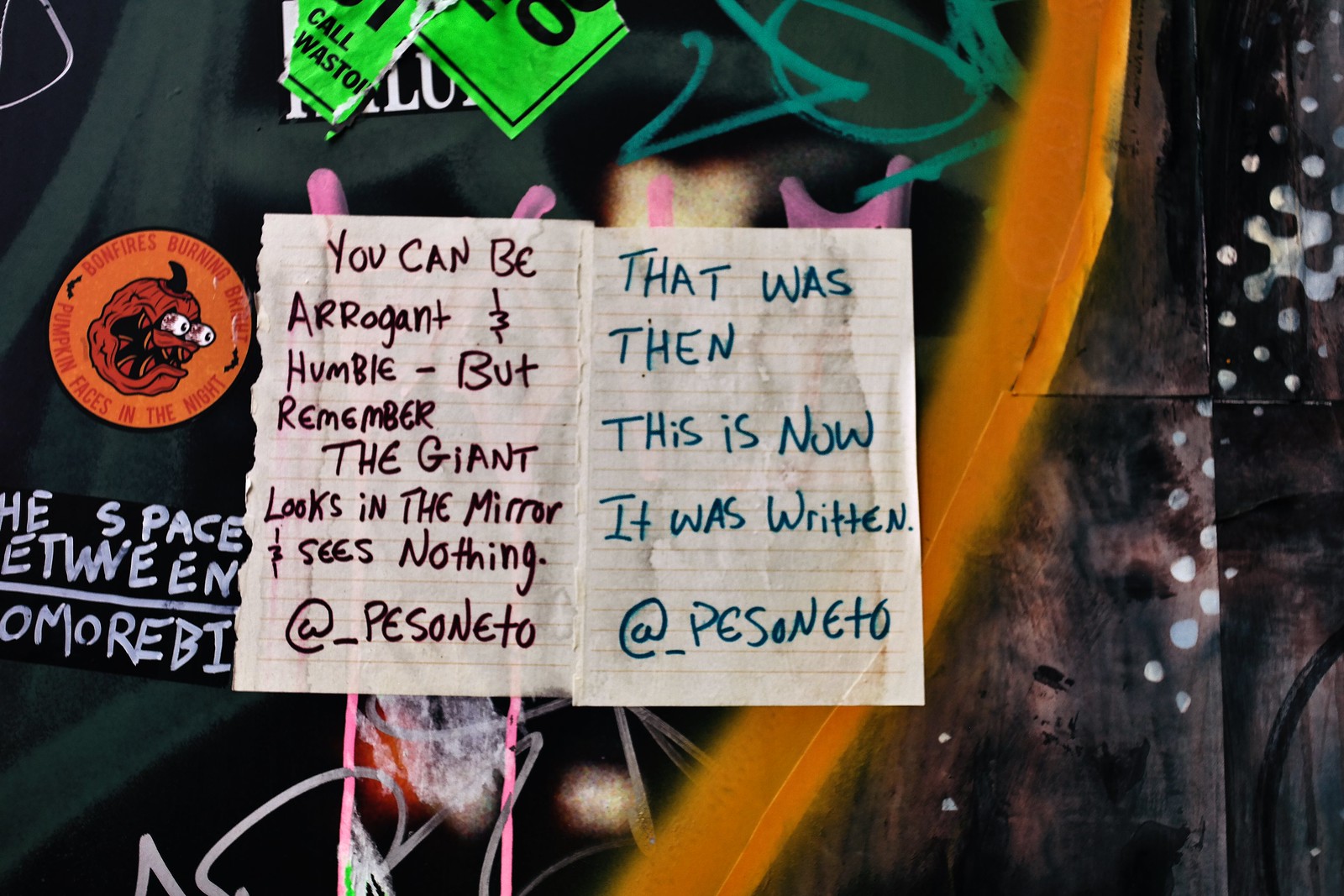The image features a dark, graffiti-covered background displaying two pieces of lined paper with tattered left edges, as if torn from a notebook. The left page, written in bold black marker, states: "YOU CAN BE ARROGANT AND HUMBLE, BUT REMEMBER THE GIANT LOOKS IN THE MIRROR AND SEES NOTHING," and is signed "@pesoneto". The right page, written in teal, reads: "THAT WAS THEN, THIS IS NOW," followed by the same signature "@pesoneto". The chaotic backdrop includes various colorful scribbles and symbols, with a notable yellow-orange button featuring a pumpkin with protruding eyes.